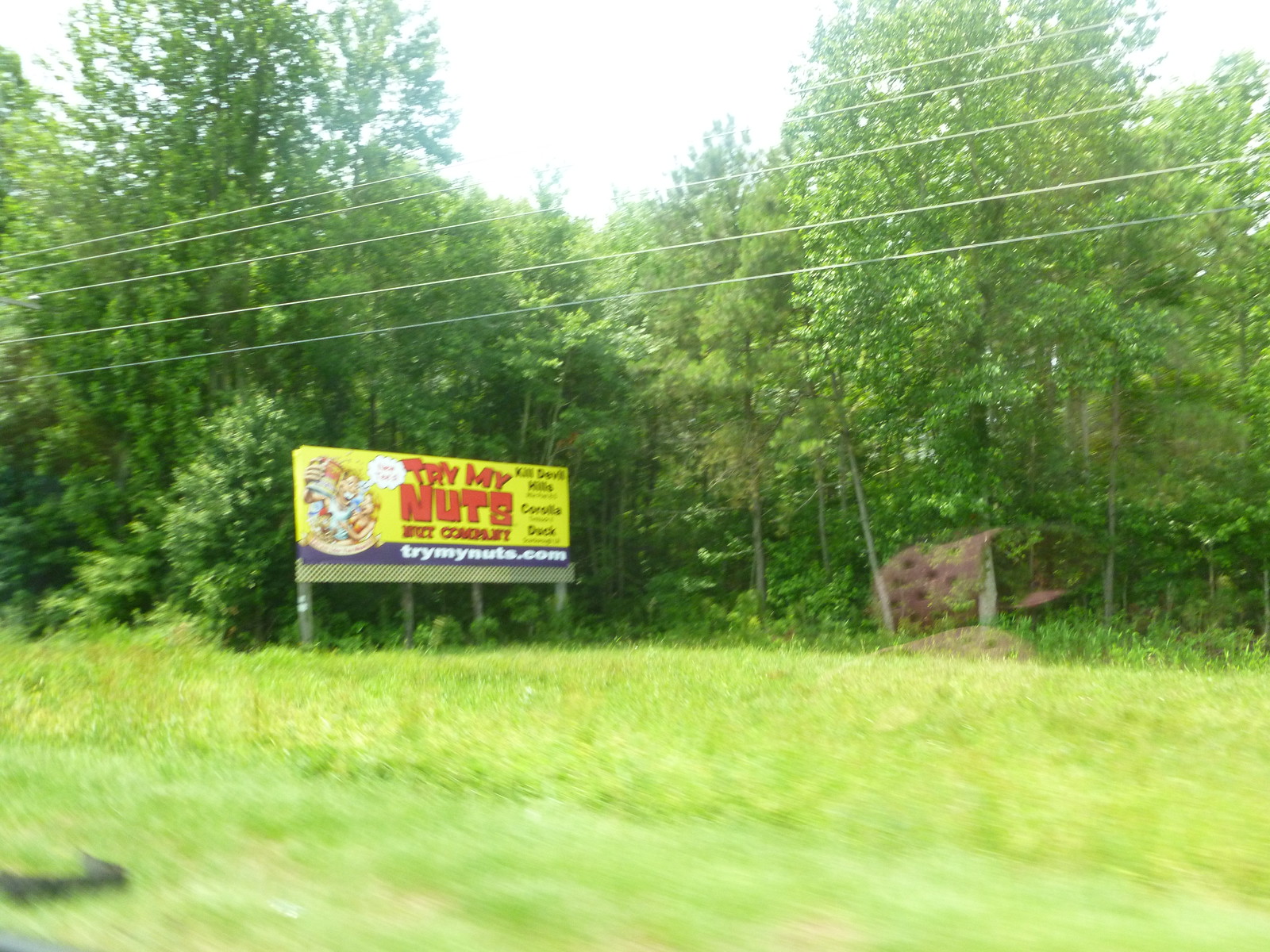The photograph captures a vivid scene through a window, overlooking a lush field of green grass and dense trees. A prominent feature in the image is a quirky billboard that humorously promotes “Try My Nuts” with the web address TryMyNuts.com. The billboard lists locations in Kill Devil Hills, Corolla, and Duck, and contains an image likely tied to the business. There are faint reflections of an interior seat on the window, suggesting the photo was taken from inside a moving vehicle, which accounts for the slight blur and visible rail lines in the foreground. The overall composition conveys a blend of nature and roadside marketing.